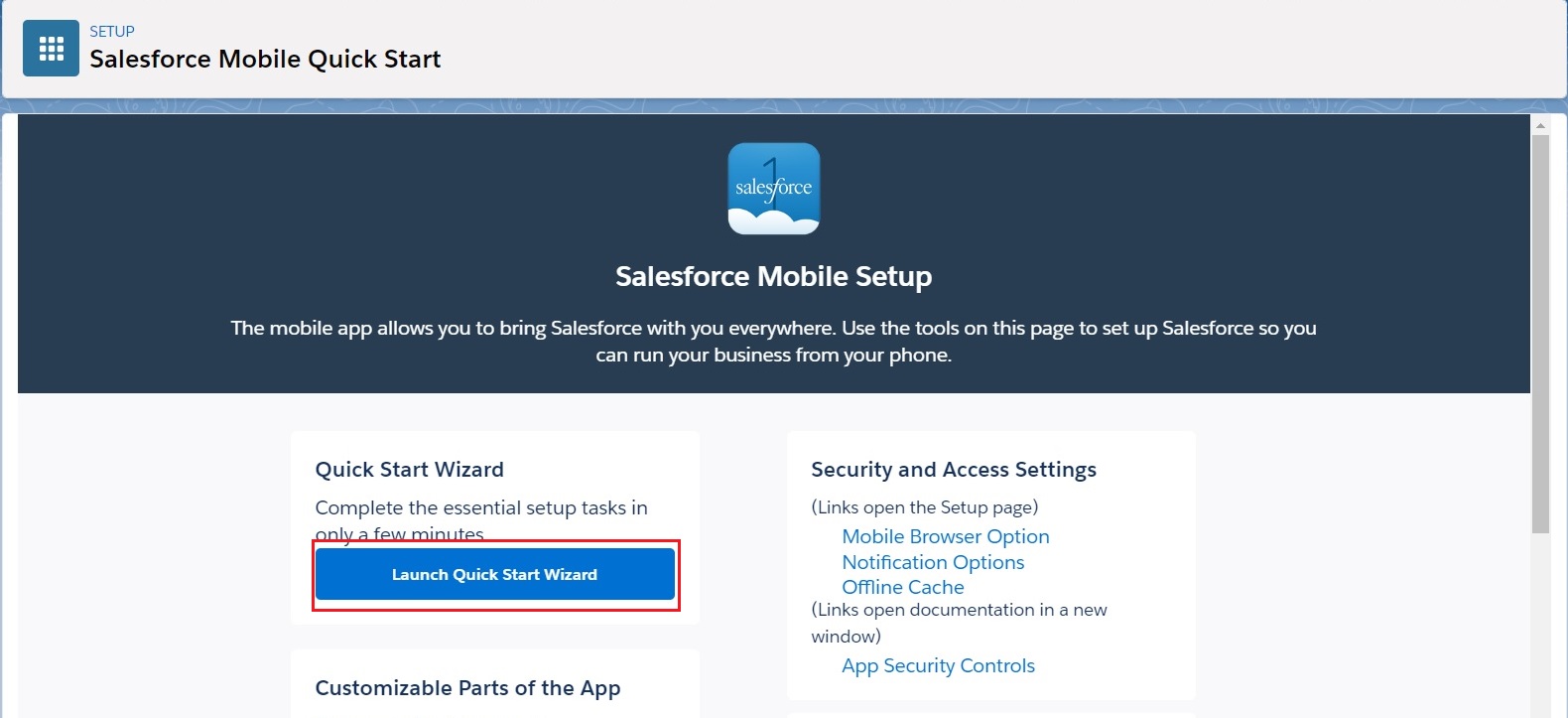**Detailed Descriptive Caption:**

The image depicts the setup menu for Salesforce Mobile Quickstart. In the upper left corner, there is a small blue box featuring keypad button icons. Adjacent to this box is a blue "Setup" button. Prominently displayed next to these elements is the title "Salesforce Mobile Quickstart" in bold black text.

Directly below the title, there's a notable blue box containing an icon of the number "1" floating above stylized clouds, with the word "Salesforce" integrated into the design. This box includes the text "Salesforce Mobile is set up" in white. The descriptive text within the blue box highlights the advantages of the mobile app, emphasizing its capability to allow users to carry Salesforce functionalities wherever they go. It suggests utilizing the tools on this page to configure Salesforce for mobile use, facilitating business operations directly from a phone.

Beneath this description, a prominent feature is a "Quickstart Wizard" button, which invites users to "Complete the essential setup task in only a few minutes." A blue bar, labeled "Launch Quickstart Wizard" in white text, is outlined by a red box indicating it is an instructional feature.

To the right, a white box encloses the "Security and App Settings" section, with several links in blue text for further configuration options: "Mobile Browser Option," "Notification Option," "Offline Cache," "Open Documents," "New Window," and "App Security Controls."

At the bottom left of the interface, another button is labeled "Customize parts of this app," allowing users to modify different aspects of the mobile application.

Overall, this setup menu is designed to guide users through the initial configuration of Salesforce Mobile, making it easier to manage their business needs on-the-go.